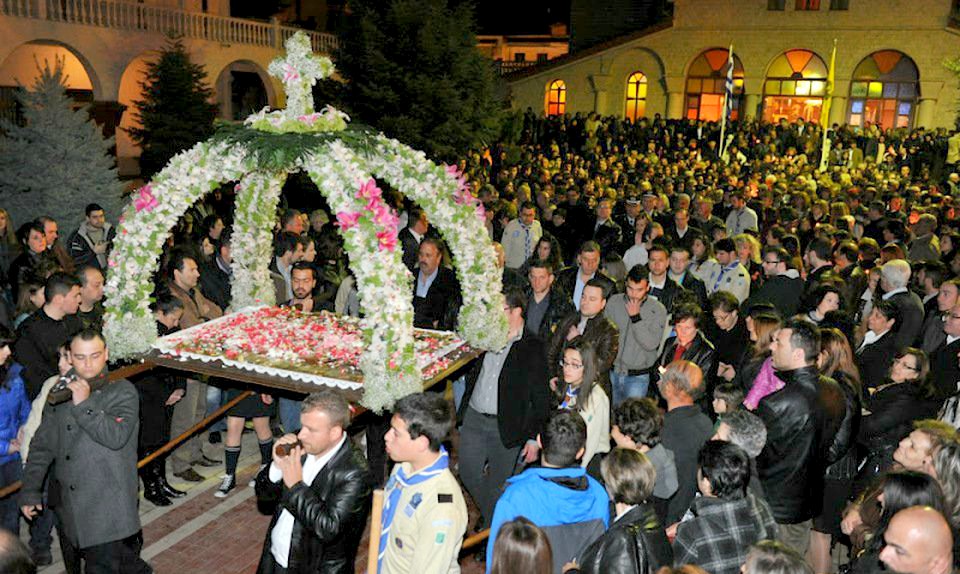In this image, a large crowd, possibly within a church courtyard or in a square outside a church, is gathered shoulder to shoulder, engulfing the scene with a vibrant mix of colors from flags waving in the background. The church building is discernible by its stained glass windows, which display intricate patterns in orange, yellow, red, and blue. Central to the crowd is a procession where four men are prominently featured—two at the front and two at the back—steadily holding long poles over their shoulders. These poles support a grand, rectangular platform adorned with an abundance of pink, white, and green flowers, meticulously arranged to form delicate arches and columns. The platform, which resembles an ornate tower or possibly even a ceremonial bier, culminates in a lush, mossy centerpiece crowned by a cross composed of green flowers. This elaborate floral display suggests it may be a part of a deeply rooted tradition, possibly a memorial or a religious celebration. The dense congregation and the solemnity in the arrangement of flowers lend a sense of reverence to the gathering, indicating it might be an event of significant cultural or spiritual importance, possibly set in a locale outside the U.S., perhaps India or another country with similar ceremonial customs.